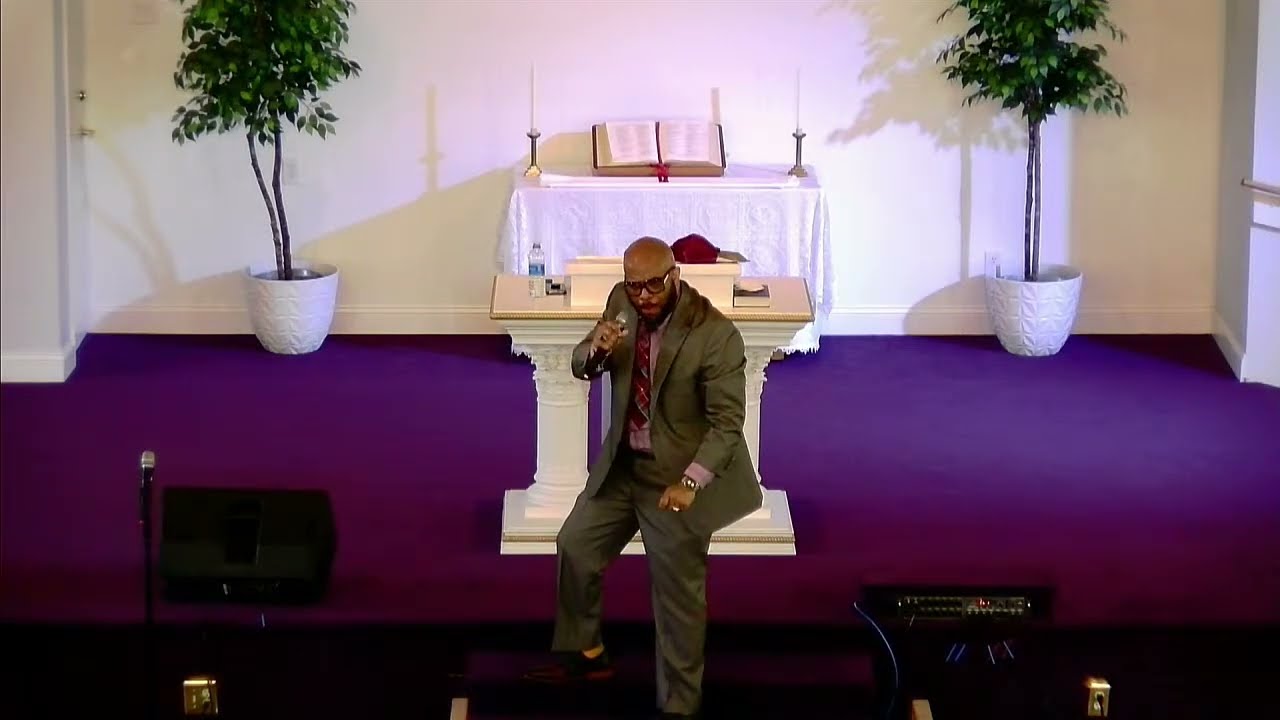The image depicts an interior church setting from a higher vantage point, looking down at a preacher addressing the congregation. The preacher, a bald black man wearing glasses with large black frames and golden arms, is dressed in a light gray suit, a light purple shirt, and a burgundy plaid tie. He is holding a silver microphone in his right hand as he stands on the steps leading up to a purple-carpeted altar. 

Behind the preacher, the altar features a purple platform with a white lectern. Further back, a raised table covered in a shiny white tablecloth holds an open book, presumably a Bible, flanked by two tall candle holders with long-stem candles. This table is set against a white wall, with large white potted plants with thin trunks and lush green leaves positioned symmetrically on each side. Additional audio equipment, including speakers and microphones, can be seen around the area.